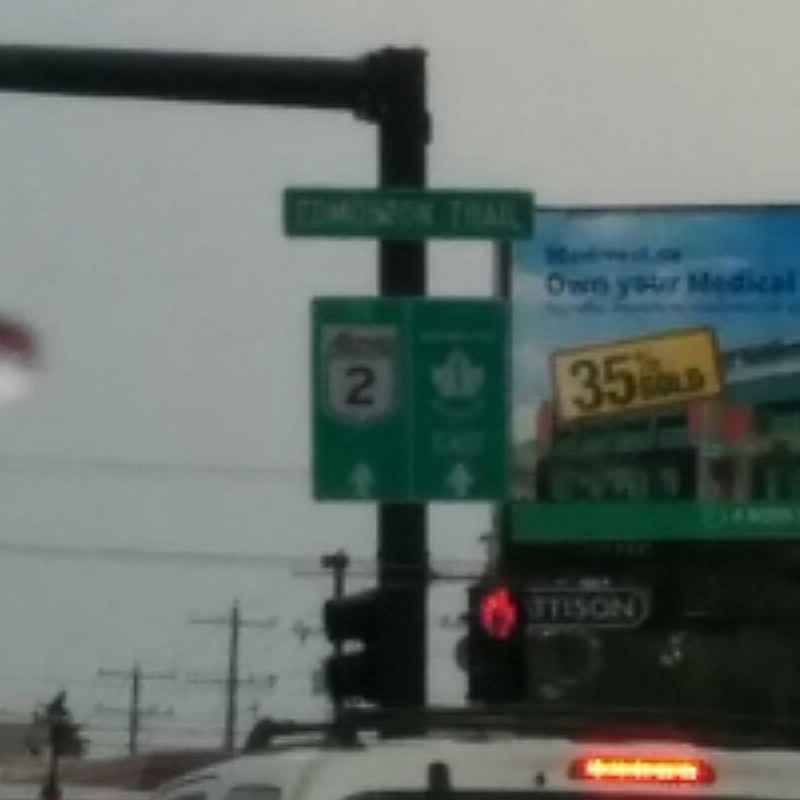This daytime color photograph captures an intersection scene under a grayish-white sky. The central focus is a large metal pole forming an upside-down, backward "L" shape on the left side of the image. This pole supports several street signs. At the top is a blurry street name, likely "Edmondson Trail." Below it, a rectangular sign prominently displays "Route 2" with a white arrow pointing forward, and beside it, another sign with a white leaf and a similar arrow.

A red traffic light is situated below these signs. To the right of the pole, a series of billboards can be seen, including one that reads "Own Your Medicine" and another stating "35 1⁄2 Sold." In the distance, electrical lines stretch across the sky.

In the lower part of the photograph, the roof of a white SUV is visible, featuring an orange taillight and a luggage rack. The entire scene is somewhat blurry, contributing to a sense of motion and activity at this busy intersection.